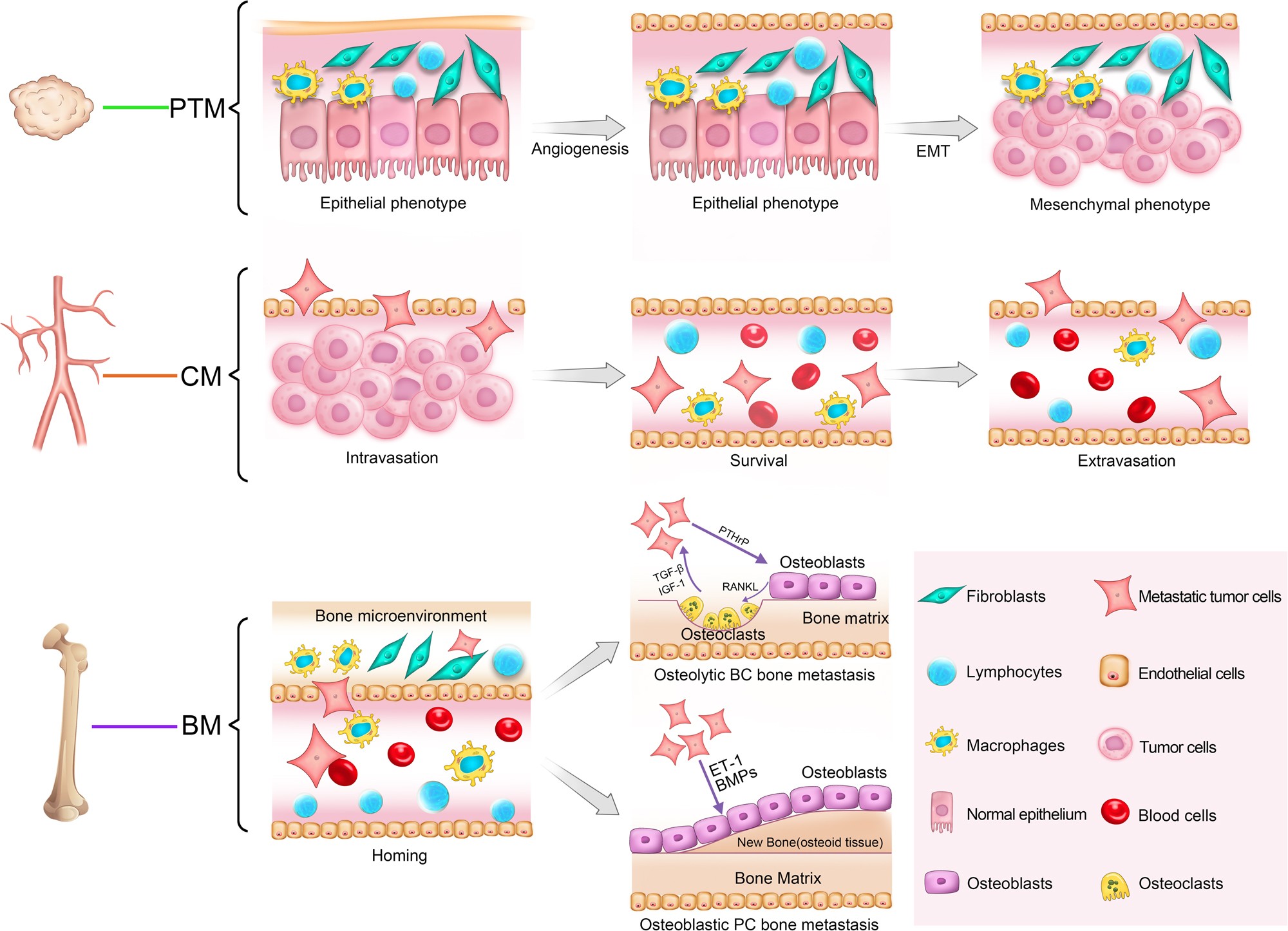The image is a schematic representation divided into three rows, each conveying a distinct stage or process.

**Top Row:**
- Contains three side-by-side images labeled as different phenotypes: "Epithelial Phenotype" on the left, "Epithelial Phenotype" in the middle, and "Mesenchymal Phenotype" on the right.
- Images are in various shades of pink, green, and yellow.
- Black text annotations detail processes: gray arrows point from the first to the second image labeled "Angiogenesis," and from the second to the third labeled "EMT."
- To the left, a bracket labeled "PTM" with a cream-colored blob is present.

**Middle Row:**
- Features three diagrams:
  - The first diagram, in pinks and yellows, is labeled "Intravasation."
  - The second diagram, adding reds and blues, is labeled "Survival."
  - The third diagram, also in reds, pinks, blues, and yellows, is labeled "Extravasation."
- A red vein is prominently visible in the center section, labeled "CM."

**Bottom Row:**
- Depicts a bone structure with the text "BM" indicating bone metastasis.
- First image in the row is labeled "Homing" with shades of green, yellow, red, and blue.
- The second image is divided into two sections:
  - "Osteolytic BC Bone Metastasis" in purples, yellows, and pinks.
  - "Osteoblastic PC Bone Metastasis" similarly colored.
- On the right, a legend explains each shape and their corresponding elements with black text.

**Legend Details:**
- Includes descriptions like fibroblasts, lymphocytes, macrophages, normal epithelium, osteoblasts, metastatic tumor cells, endothelial cells, blood cells, and osteoclasts.

The entire image is likely depicting the progression and different aspects of cancer metastasis, showing changes from epithelial to mesenchymal phenotypes, angiogenesis, intravasation, survival, extravasation, and finally, homing to and affecting bone.